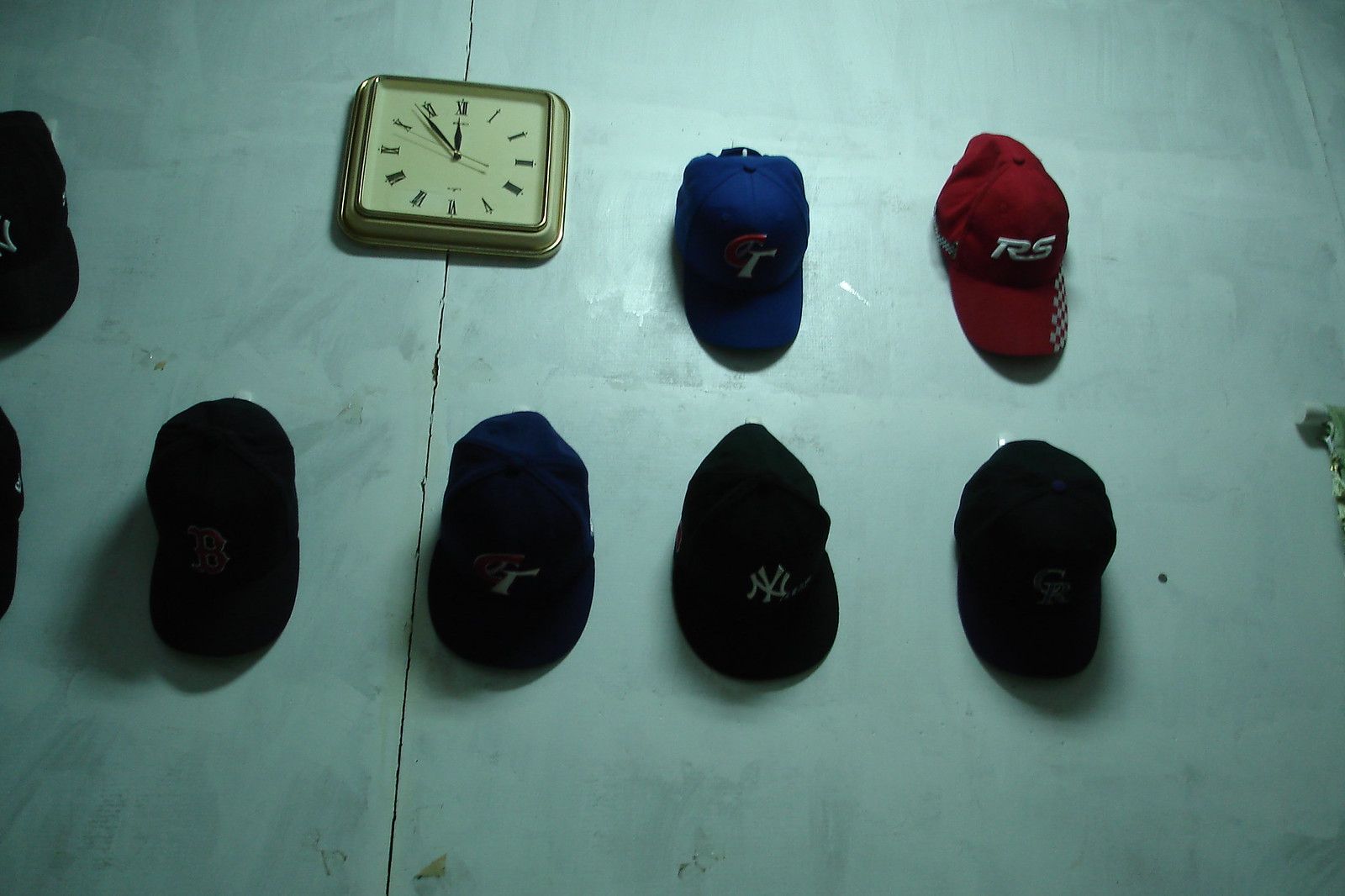A detailed color photograph captured under artificial lighting features a collection of baseball caps hanging on a dirty wall, which is painted a dusky green color with a conspicuous crack running vertically down its center. At the top of the image, centrally aligned with the crack, is a square clock with a silvery gold rim and a white face displaying Roman numerals. The clock reads five minutes to twelve. To the right of the clock hangs a red cap with white lettering that reads "RS," and to its left is a blue cap with the lettering "GT" in red and white. Below these, there is a black cap with "YN" in white and another black cap with "GR" text on the front. Further down, a blue cap identical to the one marked "GT" is visible, alongside another black cap featuring a letter "B" in red and outlined in white. Additionally, metal keys can be seen hanging on the right side of the image. The wall appears heavily stained with splotches, especially notable on the middle left and right edges, contributing to its overall grimy look.